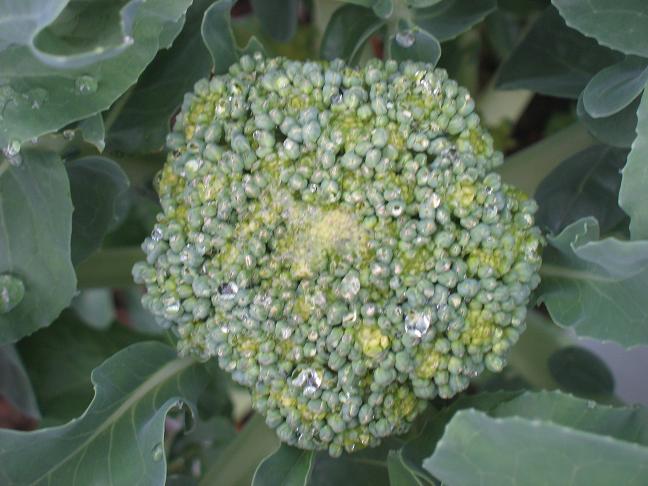This image captures a detailed, close-up view of what appears to be a head of broccoli, although its unusual coloration and texture may suggest otherwise. The core of the composition features a tight, compact bunch of small, circular dots or buds, predominantly in shades of light green, yellow, and hints of blue-green, contributing to a somewhat flower-like appearance. The buds display a mix of mint green with a whitish or ashy coating, interspersed with patches of lime green and yellow.

Surrounding this central structure are large, healthy-looking leaves that range in color from dark green to light green and bluish-green, some with noticeable water droplets on their surface indicating recent watering. The leaves take up the entire background of the image, framing the focal point of the central bud cluster. The head of broccoli appears slightly dusty or crystallized in some areas, adding to its intriguing texture.

Though it resembles broccoli, the atypical colors—light blue, yellow, and various greens—suggest it might be either maturing, affected by its environment, or even possibly another plant in the same family. Overall, the image presents a rich, intricate view of a plant head surrounded by lush leaves, offering a complex interplay of color and texture.